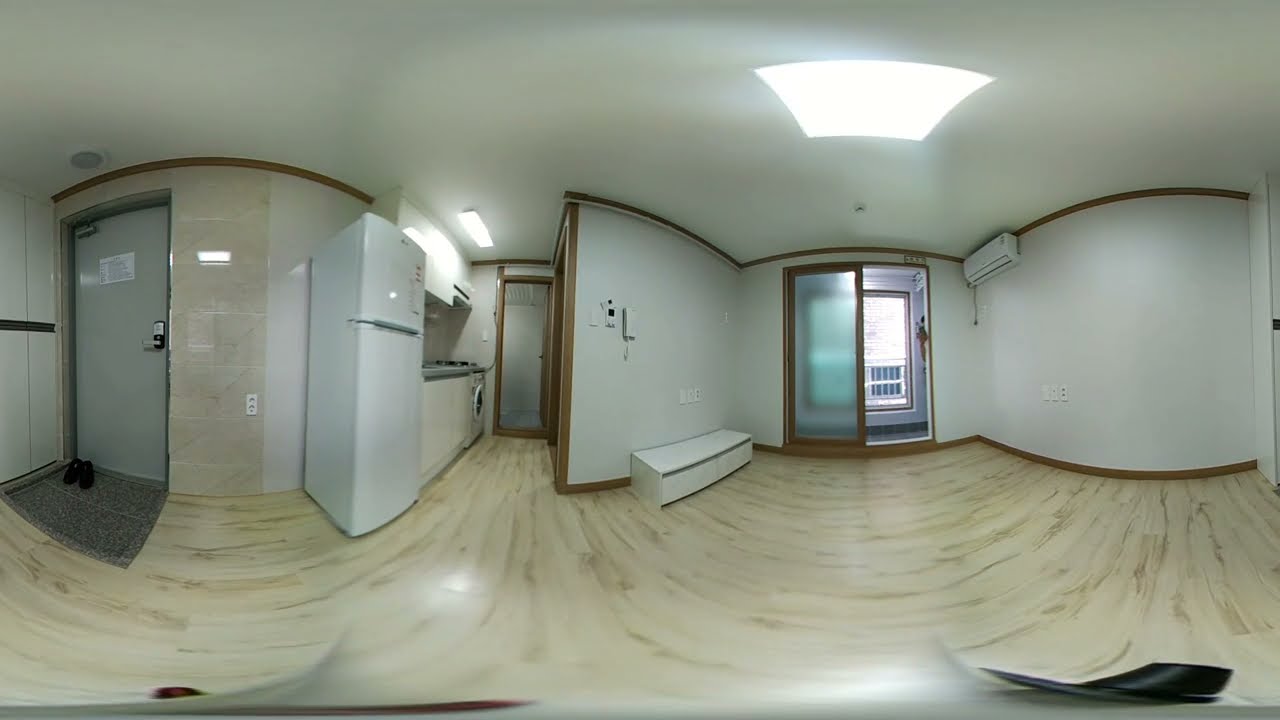This panoramic image depicts a mid-day scene inside a small, sparsely furnished apartment. Predominantly, the space features light brown hardwood flooring that extends throughout. On the far left, there's a heavy, light gray metal door equipped with a keypad. In front of the door, a dark gray mat hosts a pair of black shoes. Adjacent to the door, the floor transitions to glossed light brown tiles.

To the immediate right of the door lies the kitchen area, which includes a tall, white, American-style refrigerator, a range with an overhead vent, and cream-colored cabinets. A washing machine is positioned at the far end by the wall. Above, a light fixture illuminates the kitchen space. 

Dominating the center foreground, a long rectangular white cabinet or TV stand with drawers is positioned against a white wall equipped with a phone and various electrical outlets and plugs. Nearby, an air conditioning unit is mounted on the top left corner of the right wall. 

To the right, a narrow wooden-framed doorway leads to another room. Directly ahead, there’s a sliding glass patio door with frosted glass on one side, opening onto a balcony that provides a view of another building. The ceiling is white, featuring a prominent square light on the right side, casting a bright glow over the living space. No text is visible within the image, and the primary colors include shades of white, off-white, brown, silver, gray, and light blue.